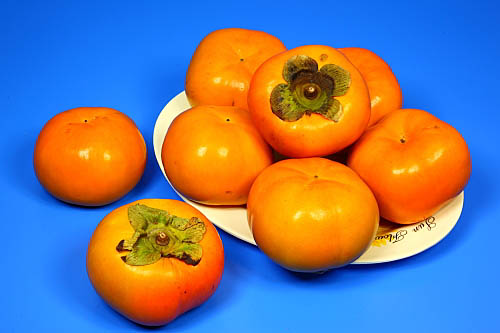The vibrant color photograph is set against a bright blue background and features a white, round or oval plate possibly made of china or plastic. The plate, which has the black writing "Sun Florida" on it, holds an array of six orange persimmons, arranged in a circular, flower-like shape around the plate's edge. Each of these persimmons is primarily face down, with their stem sides up, except for the one in the center, which has its stem side facing upwards. The central persimmon displays signs of decay with a discolored greenish-brown stem, hinting at rot spreading from the center outward. 

To the lower left of the plate, two more persimmons rest on the table. The upper one is stem-side down, casting a slight shadow, while the lower one, similar to the central persimmon, has a stem-side up and shows signs of decay with a grayish-green discoloration around the stem area. The persimmons on the plate exhibit hues ranging from orange to yellow and reddish, with their large, flower-like green and brown stems adding to the detailed and slightly decaying appearance of the fruits.